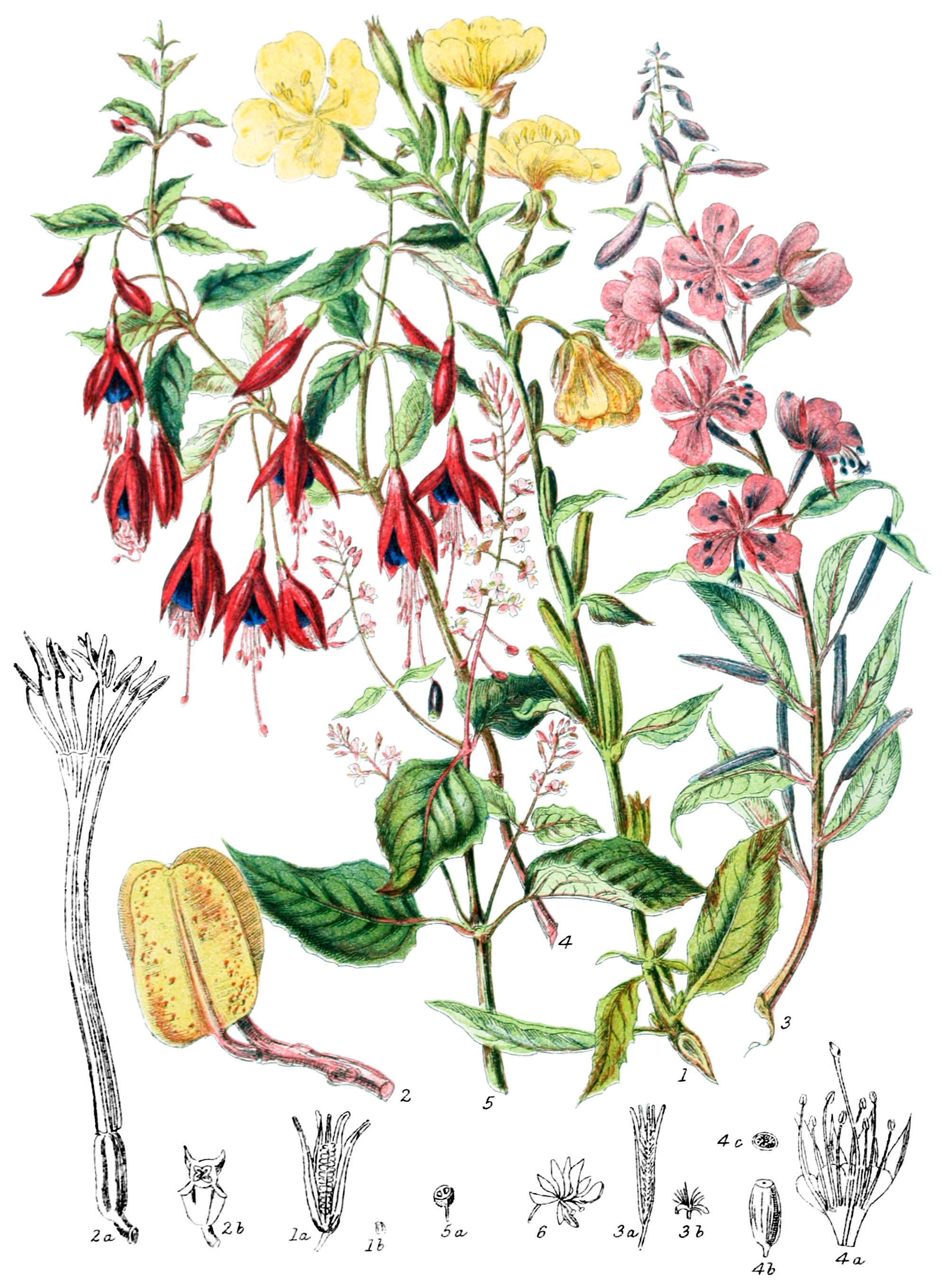The botanical illustration is set against a solid white background, which takes up the major portion of the canvas. The artwork features an array of flowers with flowing, delicate petals and long green stems adorned with green leaves. The illustrated flowers come in various vibrant colors, including pink, yellow, red, and lavender. Notably, there are pink flowers with long brown stems, yellow flowers with green leaves hanging off their stems, and droopy red flowers with blue seeds inside. Along the bottom of the illustration, there are additional elements depicting different forms, such as a bulbous yellow flower and black and white sketches that resemble parched flowers, labeled with numbers and letters. This color pencil illustration includes whimsical flower shapes, with some resembling an owl, freshly picked corn, a seed, a tall tulip, and a small weed, all meticulously drawn and detailed.